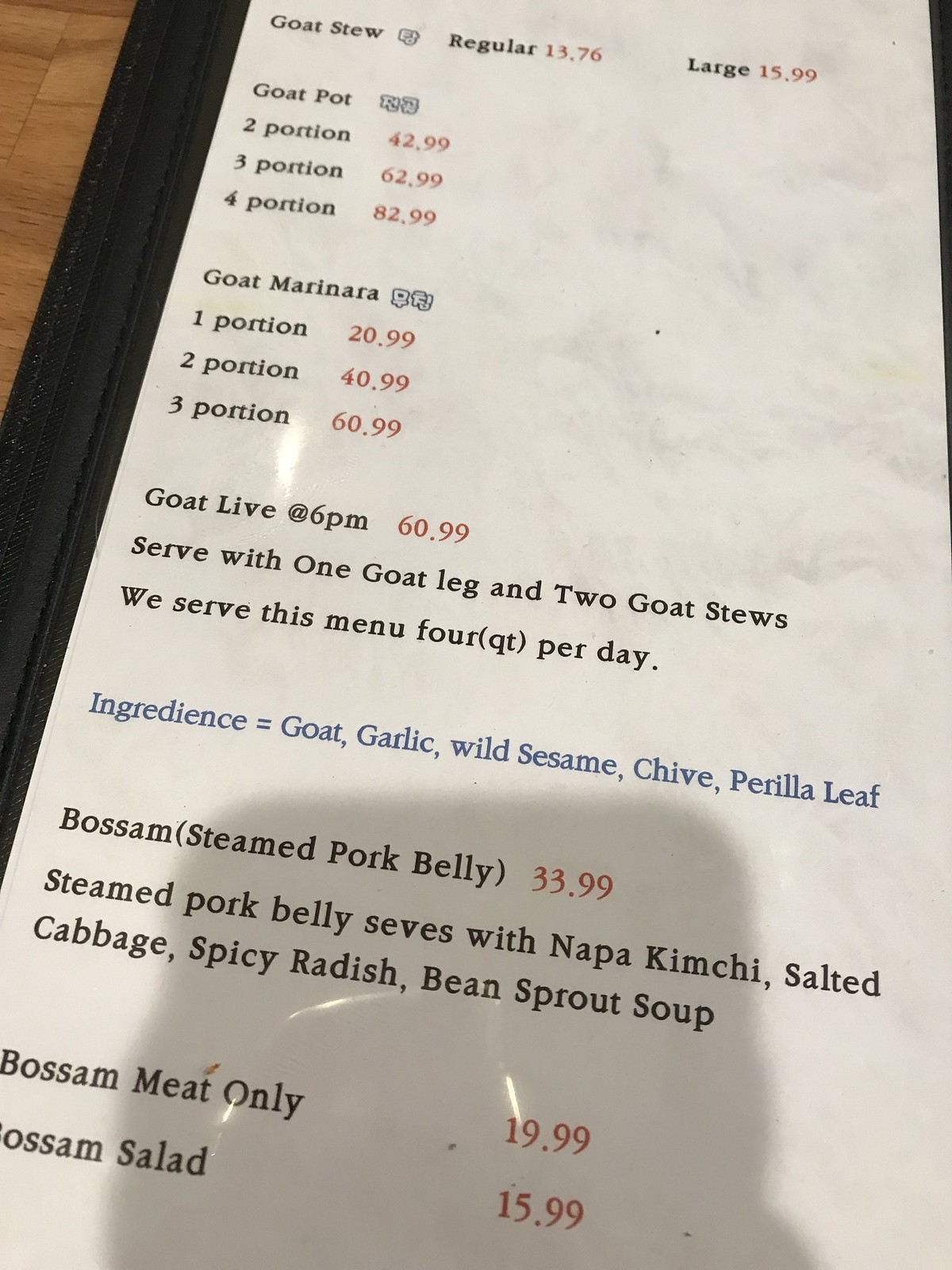The image depicts an open, tall, rectangular menu, bordered in black leather, likely for a restaurant. The inside page displayed has a white background with the various dishes and their prices neatly listed in both black and red text:

1. **Goat Stew**
   - Regular: $13.76 (in red)
   - Large: $15.99 (in red)

2. **Goat Pot**
   - Two portions: $42.99 (in red)
   - Three portions: $62.99 (in red)
   - Four portions: $82.99 (in red)

3. **Goat Marinara**
   - One portion: $20.99 (in red)
   - Two portions: $40.99 (in red)
   - Three portions: $60.99 (in red)

4. **Goat Live@ 6 p.m. ** 
   - $60.99 (in red)

   Notes: **Served with one goat leg and two goat stews.**

5. **Bosam** (Steamed Pork Belly)
   - $33.99 (in red)
   - Description: **Steamed pork belly served with kanapa kimchi, salted cabbage, spicy radish, and bean sprout soup.**

6. **Bosam Meat Only**
   - $19.99 (in red)

7. **Bosam Salad**
   - $15.99 (in red)

A note in blue font at the bottom of the menu reads: **Ingredients = goat, garlic, wild sesame, chive, and perilla leaf.**

The menu rests on a light brown wooden table, visible on the upper left-hand corner. There is a faint shadow at the bottom of the page, resembling the shape of a phone, suggesting the photo was taken by someone holding their phone above the menu.